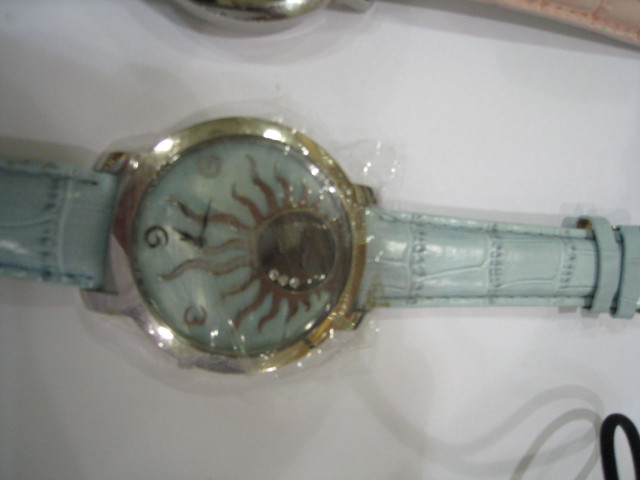In this image, we see a detailed close-up of a wristwatch set on a white surface. The watch has a mint green, snakeskin-patterned band, partially covered in plastic. The band appears to be made of leather, evident from the imprints shown on it. The circular face of the watch is encased in gold and is also covered with a thin plastic wrap. The face itself is light gray, featuring a unique design of a dark brown, multi-legged creature or abstract sunburst with a rugged pattern, which might resemble an octopus. This design has intricate rays extending outward, and part of it contains diamond chips on the right side. On the watch face, the numbers 12, 3, 6, and 9 are visible within this central design, but their positions appear slightly off, possibly due to the artistic placement or the angle of the image. Above the main watch, there is a glimpse of another watch with a pink band and a silver face. In the lower right corner, a black strap, perhaps another accessory, is noticeable, adding to the intricate composition of the image.